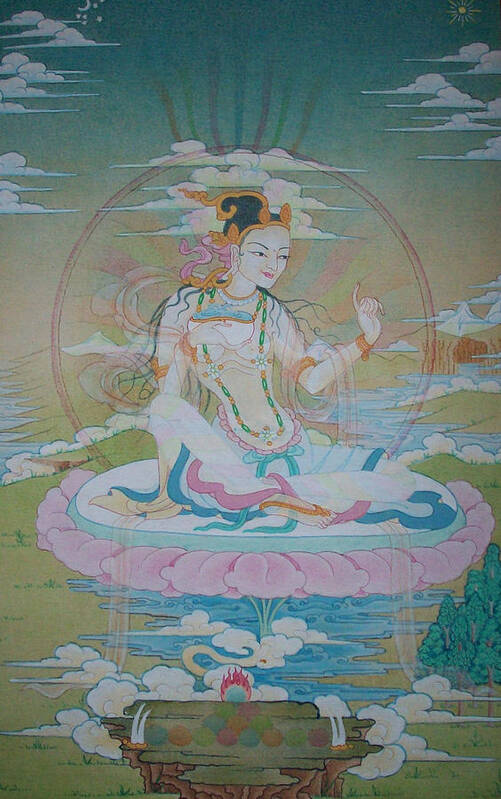In this pastel abstract illustration, an ethereal Asian or Indian woman, possibly depicted as a deity, hovers gracefully above a vibrant scene of colorful wooden planks and natural landscapes. She is seated in a cross-legged position on a cushion with a pink outer edge and a green and white center that floats in mid-air. The woman's long, flowing outfit displays an intricate mix of pastel shades—tan, pink, and blue—blending into the hues around her, making it difficult to discern where her garments end and the background begins.

Her black hair is adorned with an ornate yellow or gold headpiece, exhibiting intricate scrollwork and giving her an aura of divinity. Additionally, she wears a striking necklace of green, orange, and white flowers alongside a white and orange choker. The detailed golden headpiece complements her bare upper body and the billowing blue pants she wears. Her pose is serene, focusing intently on her left hand, which is raised slightly with a bent elbow and a clenched fist.

In the backdrop, the sky transitions from multi-green shades at the top to softer tones of beige and light pink as it descends, with wisps of clouds framing the scene on either side. The lower part of the image showcases a varied terrain including grassy hills, mountains, and flowing water streams. At the bottom, outlines of grass and a brown and dark green object are visible, along with trees to the right, enhancing the natural setting's complexity. Overall, this enchanting image merges a divine presence with a mystical landscape, creating a dreamlike and atmospheric portrayal.